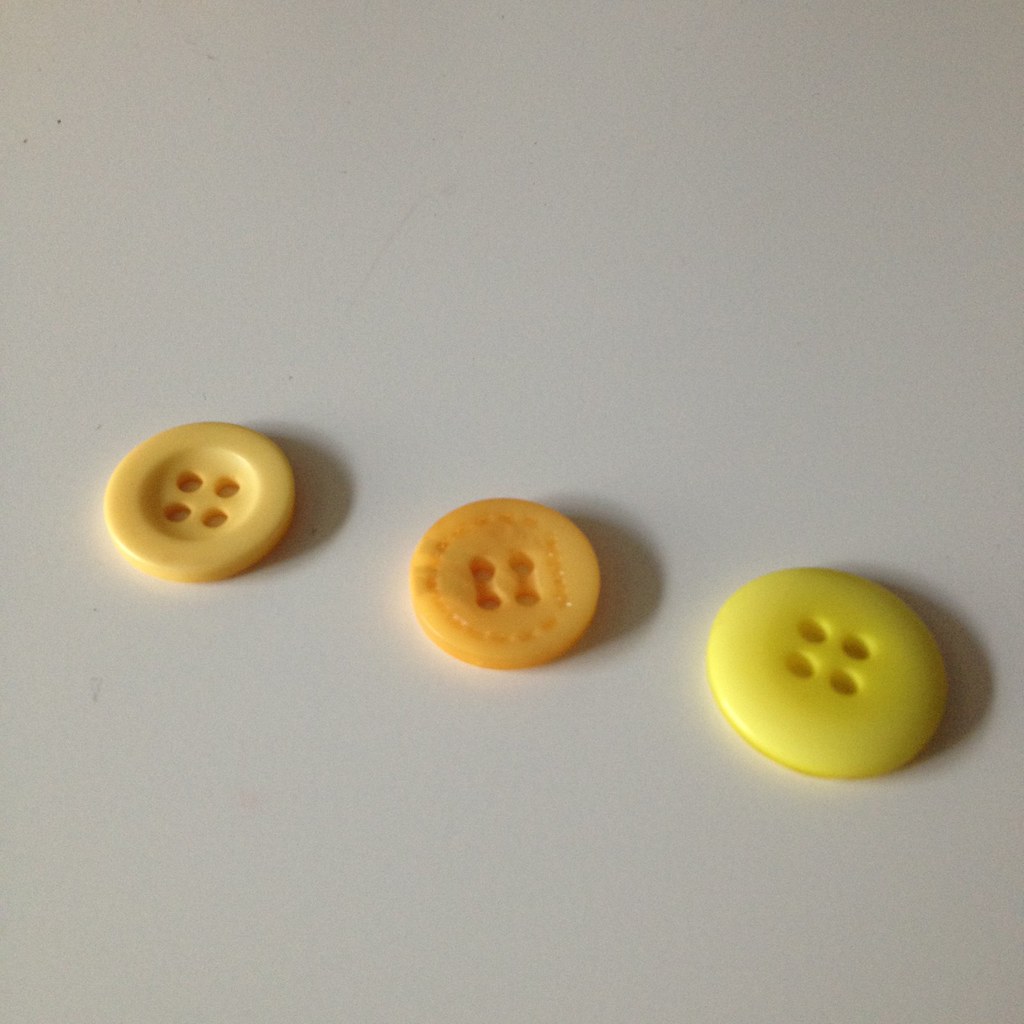This is a close-up image of three circular buttons laid on a white background, positioned in a slight diagonal from the upper left to the bottom right. The button on the upper left is tan, featuring a bowl-like indentation around its four central holes. Below and to the right is a slightly smaller orange button with textured ridges encircling its four holes. The largest button, located further to the bottom right, is a smooth, pale yellow dome with four holes. All buttons showcase distinct designs and sizes, capturing a simple yet detailed composition.